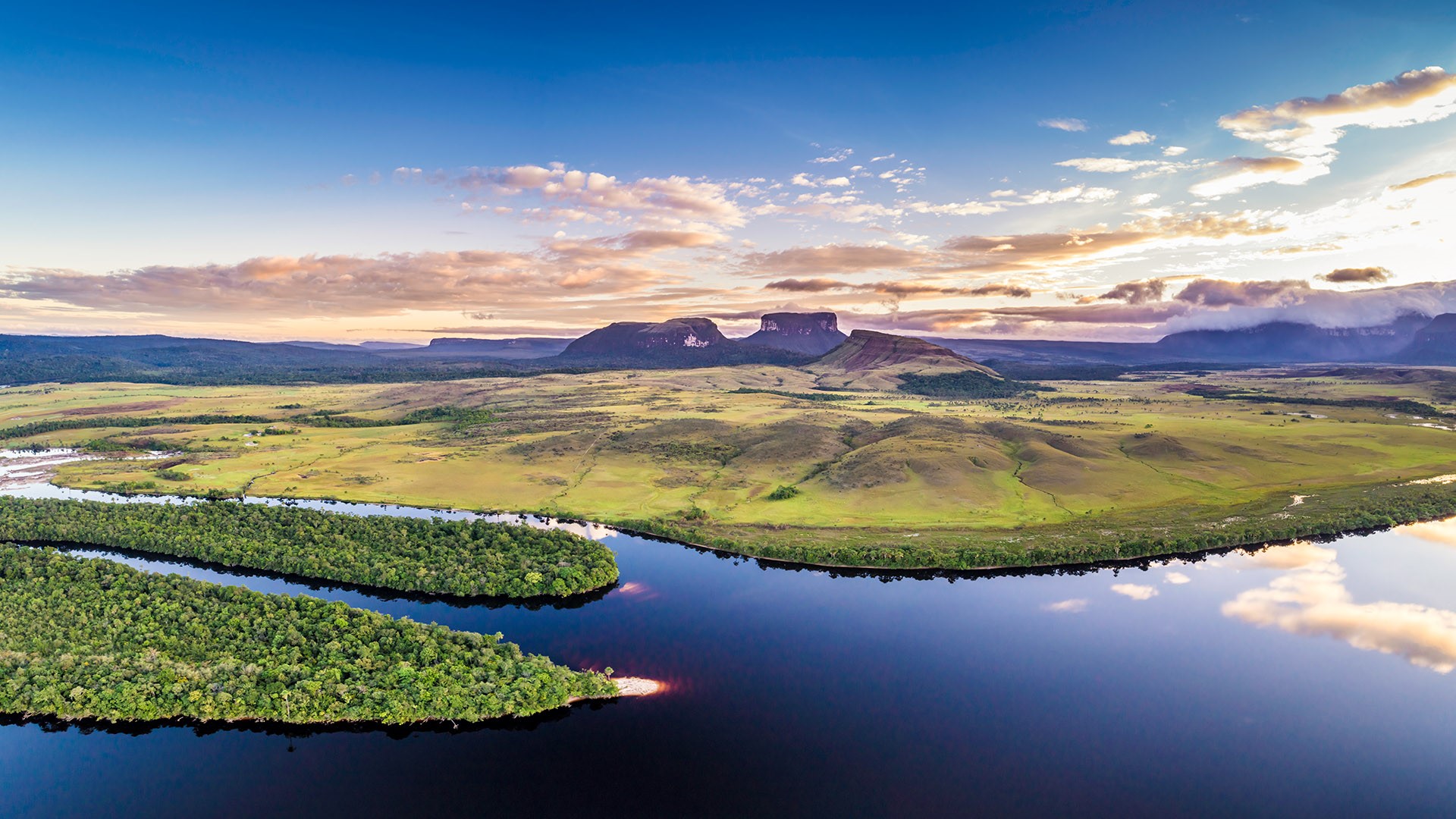This image presents a breathtaking panoramic landscape featuring a crystal blue body of water that mirrors the sky and clouds, creating a serene and almost ethereal scene. To the left, green and brown highlands and peninsulas stretch out, covered in dense, healthy vegetation with vibrant greenery, suggesting lush forests. These landmasses split the water, forming islands and adding to the picturesque vista. In the midground, smooth and calm water enhances the reflections, making the clouds appear as though they are part of the lake. The distant background showcases a blend of green fields and flat mountain areas, which take on a grayish-purplish hue, suggesting a backlit setting sun. The overall scene portrays a tranquil delta region with diverse terrain, from verdant peninsulas and grassy fields to distant rock formations, evoking a sense of expansive, untouched natural beauty.